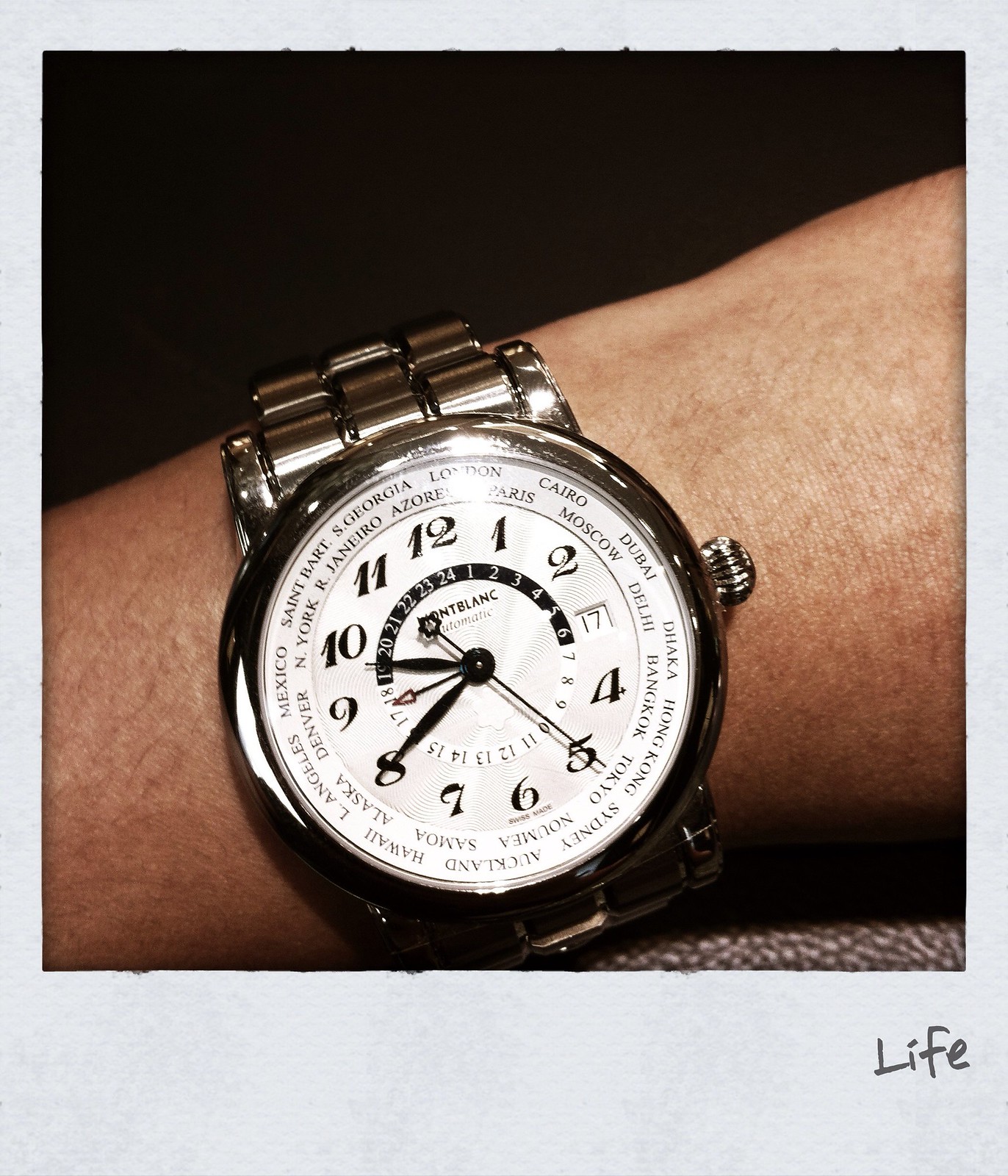The image depicts a wristwatch on a man's arm, presented in what looks like an old Polaroid photograph with a distinctive white border. In the bottom right corner of this border, the word "Life" is hand-written in black ink. The arm, positioned diagonally from the lower left to the upper right, shows some black hair and varying skin tones—lighter on the right and tanner on the left. The watch itself is entirely silver, featuring a round, silver rim and a metal bracelet composed of several jointed pieces. The watch face is white with black Arabic numerals and black hands, with smaller hands included. Surrounding the face are names of various cities such as Moscow, Cairo, London, and Hong Kong, indicative of an additional timekeeping feature. The background of the photo includes a black section in the upper left and a textured grey shadow in the lower right. The time shown on the watch is approximately twenty minutes to ten.